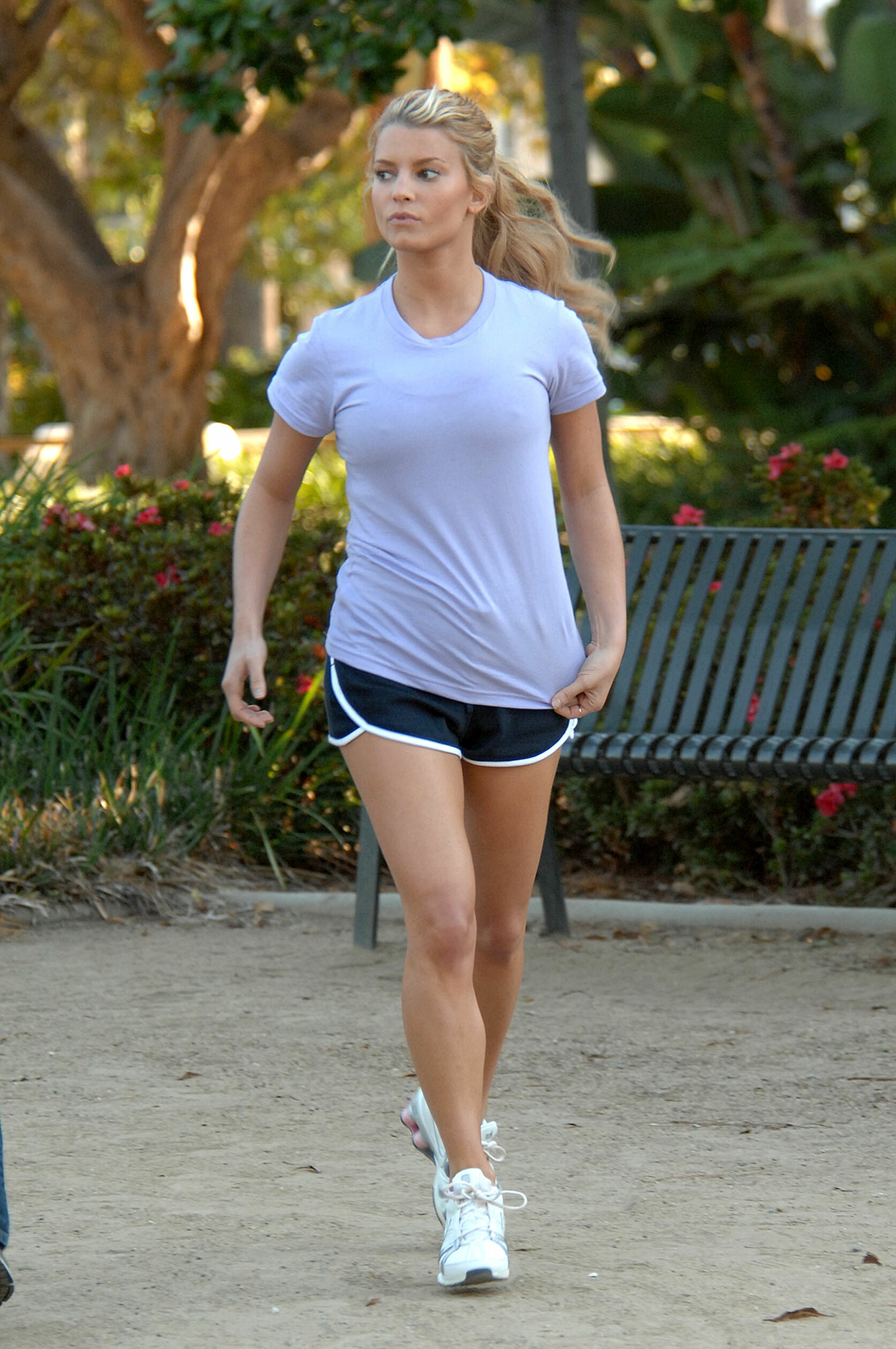In this color photograph, we see a young woman who closely resembles Jessica Simpson, prominently positioned in the mid-ground of a sunny park scene. She has blonde hair pulled back in a ponytail and is looking to her right, while her left hand clutches her gray T-shirt. She is dressed in black-blue shorts with white piping, a gray T-shirt, and white running shoes. The surface she is walking on appears to be light-colored dirt or hard-packed sand. To her right stands a green metal park bench on the sandy path. Behind the bench is a row of bushes with vibrant red or pink flowers, extending to the left. Further in the background, softened in focus, are tall trees, including some palm trees. The sunlight illuminates patches of the scene, creating a warm, inviting atmosphere.